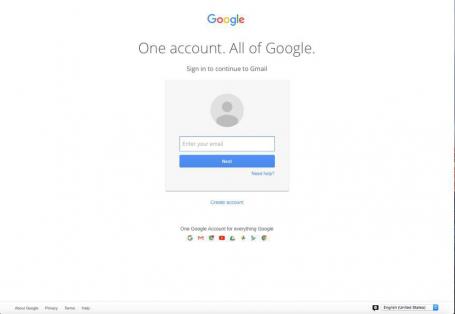This is a screenshot of the Google sign-in page. At the top center, the page features the iconic Google logo, with each letter in the familiar blue, red, yellow, and green colors. Below the logo is a line of text that reads "One account. All of Google." in gray. Next, another centered line of text states "Sign in to continue to Gmail."

Further down, there is a square gray box with a circular icon depicting a generic human figure at the top. Beneath this icon is a text box labeled "Enter your email." Situated below this input box is a prominent blue button with "Next" centered in white text.

Additionally, at the bottom of the gray box, also centered, is an option that reads "Create account." Below this, there is another line of text stating "One Google Account for everything Google." At the very bottom of the page, a series of icons representing various Google services, including Google, Gmail, and YouTube, are displayed.